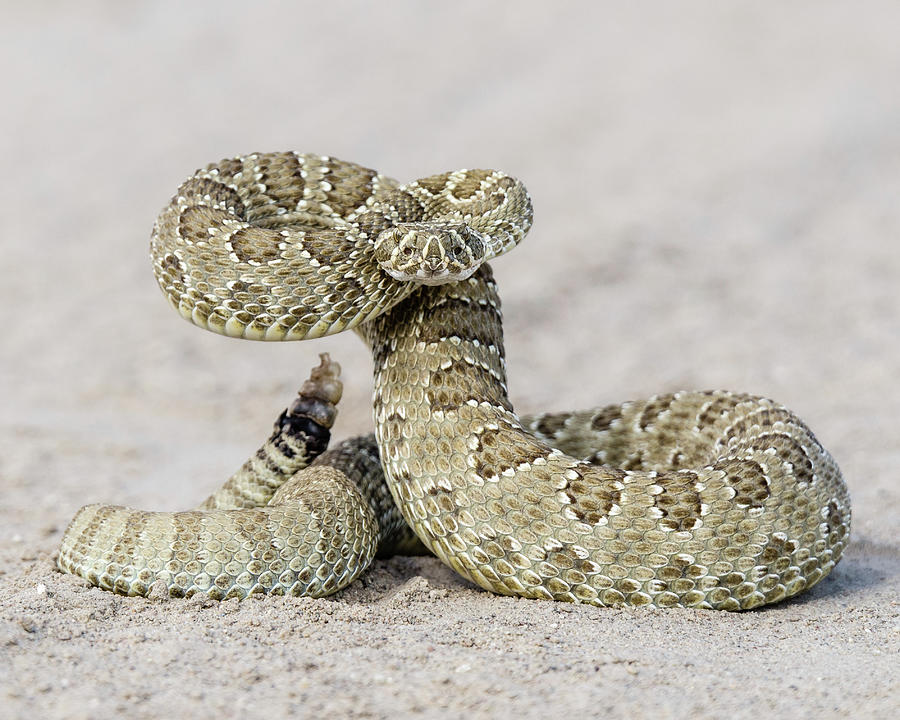This detailed caption combines all shared and repeated aspects from the descriptions:

This square-shaped photograph features a coiled rattlesnake on a fine gray sand surface sprinkled with various larger pebbles of different colors. The snake, predominantly tan with white circles filled with brown spots, has distinct dark brown partial stripes and is sharply in focus against a blurred background. The snake’s tail, adorned with a semi-transparent, brown rattle, is coiled on the left side, while its body spirals in the opposite direction in the center before rising up. The triangular head, marked by black eyes, is raised and seems to be staring directly into the camera, suggesting a poised and potentially striking stance, highlighting the snake's dangerous nature.